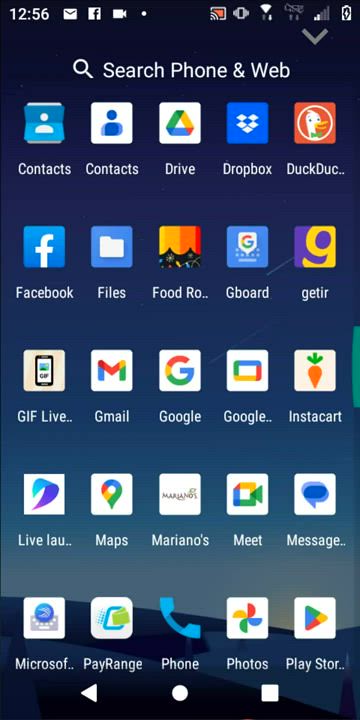A screenshot of a smartphone's home screen interface features an array of diverse app icons organized in a grid layout. At the top, a magnifying glass icon signifies the "Search phone and web" function. Below this search bar, numerous app icons are visible, including Contacts, Google Drive, Dropbox, DuckDuckGo (partially obscured), Facebook, Files, an unspecified food-related app (partially obscured), Gboard, Getter, a GIF-related app, Gmail, Google, another Google-related app (partially obscured), Instacart, an app labeled "Live," another labeled "LAU" (partially obscured), Maps, Mariano's, Google Meet, Messages, a partially obscured Microsoft app, PayRange, Phone, Photos, and the Play Store (partially obscured).

The majority of these icons are displayed with a white background and distinct symbols, while a few appear in blue with various designs. At the bottom of the screen, navigation buttons include a white circle for the Home function, a left-pointing triangle for the Back function, and a white square for recent apps.

The status bar at the top of the screen shows the current time and several notification icons, such as a letter, Facebook, camera, white dot, and a recording indicator. Additional icons on the right side of the status bar display mobile reception strength and charging status, indicating that the device is currently connected to power.